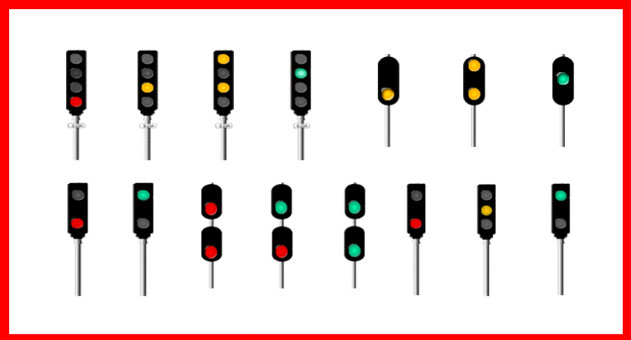The image features a detailed drawing on a white piece of paper with a red border, depicting an assortment of traffic light-like indicators. Each unit has a black rectangular housing with various light configurations and is supported by a silver rod. Here's a breakdown of the traffic light indicators from top to bottom, left to right:

**Top Row:**
1. A black rectangle with four lights: the bottom light is red.
2. A black rectangle with four lights: the second light from the bottom is yellow.
3. A black rectangle with four lights: the top light and the second light from the bottom are yellow.
4. A black rectangle with four lights: the third light from the bottom is green.
5. A black pill-shaped unit with three lights: the bottom light is yellow.
6. A black pill-shaped unit with three lights: the top and bottom lights are yellow.
7. A black pill-shaped unit with three lights: the middle light is green.

**Bottom Row:**
8. A black rectangle with three lights: the bottom light is red.
9. A black rectangle with three lights: the top light is green.
10. A black rectangle with two lights: the bottom light is red.
11. A black rectangle with two lights: the top light is green.
12. A black rectangle with a single light housing: the bottom light is red.
13. A black rectangle with a single light housing: the bottom light is green.
14. A black rectangle with a single light housing: the bottom light is green.
15. A black rectangle with three lights: the bottom light is red.
16. A black rectangle with three lights: the middle light is yellow.
17. A black rectangle with three lights: the top light is green.

This collection of traffic light indicators varies in shape and configuration, each exhibiting a unique pattern of illuminated lights in red, yellow, and green combinations.